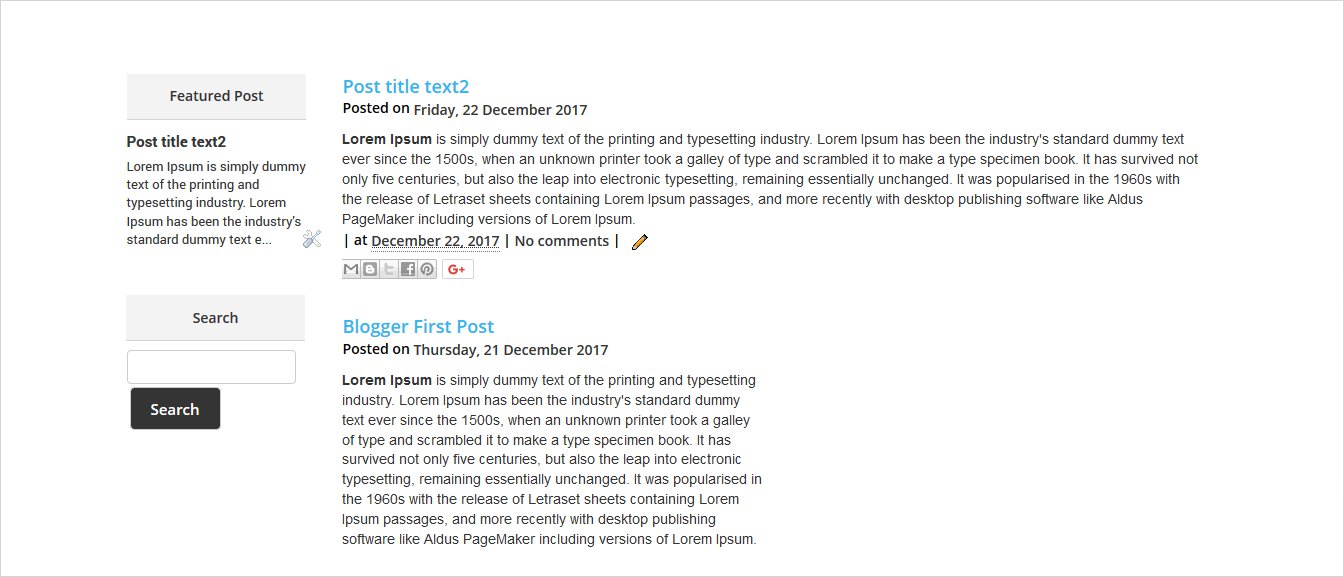The image captured from a computer screen features a detailed digital post. The highlighted section of the screen shows a featured post titled "Post Title Text 2" which was published on Friday, December 22, 2017. The text of the post includes a placeholder paragraph containing "Lorem Ipsum," a standard filler text used extensively in the printing and typesetting industry since the 1500s. The paragraph explains the historical significance and consistent usage of Lorem Ipsum, noting its persistence through five centuries and adaptation into electronic typesetting. It was notably popularized in the 1960s with the release of Letraset sheets and later with desktop publishing software such as Adels and PageMaker.

Below the featured post, there is another entry titled "Blogger First Post," which was published a day earlier, on Thursday, December 21, 2017. This post appears to share similar content about Lorem Ipsum, reinforcing the idea that the text might be repurposed for another blog post. The repetitive use of this placeholder text indicates a potential draft or template being prepared for future posts. The overall screen presents a snapshot of a blog's editorial timeline, capturing the ongoing process of content creation and publishing.